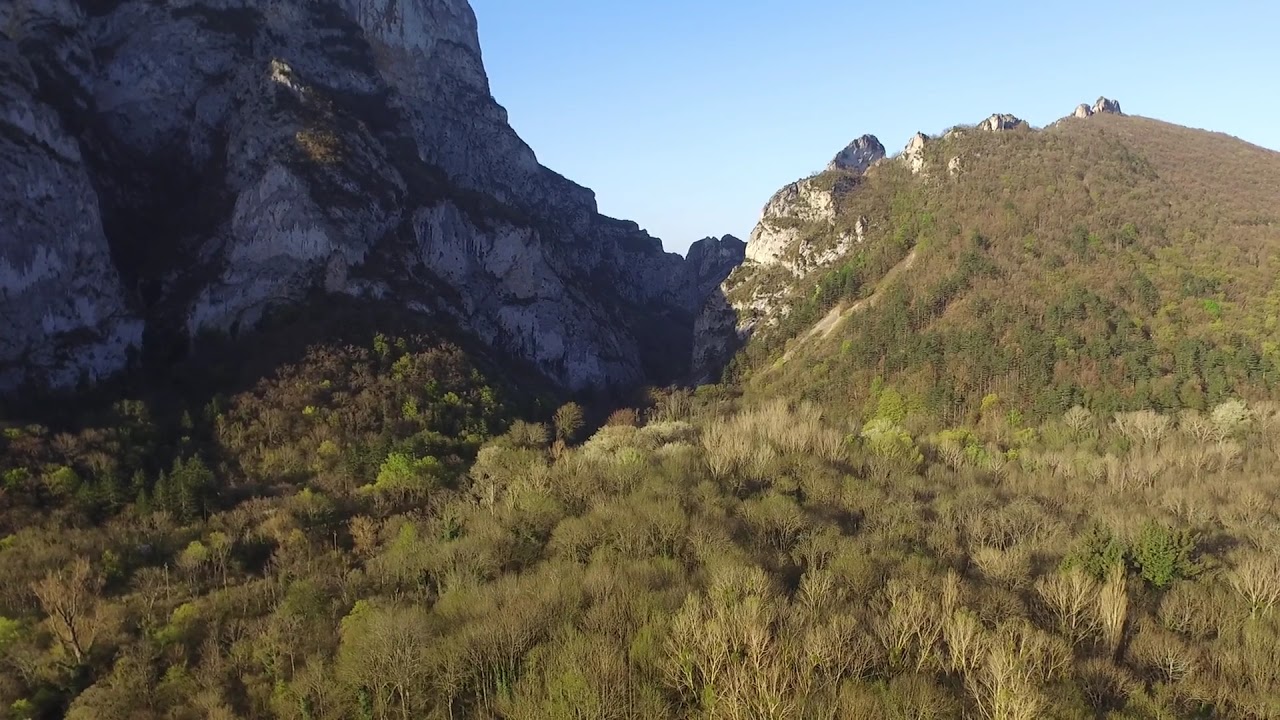This picturesque landscape photograph captures a striking contrast between rugged mountain terrain and lush foliage on a clear, sunny day. Dominating the left side of the image, a steep and shadowed rocky mountain cliff extends from the midpoint to the top left corner, characterized by dark blues and grays with sparse black patches of foliage. In the foreground, a gently sloping valley covered with dense trees stretches from the halfway mark on the left to about three-quarters up the right-hand side, showcasing a transition to more autumnal hues with hints of red and brown amidst the diminishing greens. The scene is encapsulated by a vibrant, cloudless blue sky occupying the upper right corner, adding a serene backdrop to the vivid natural tableau.